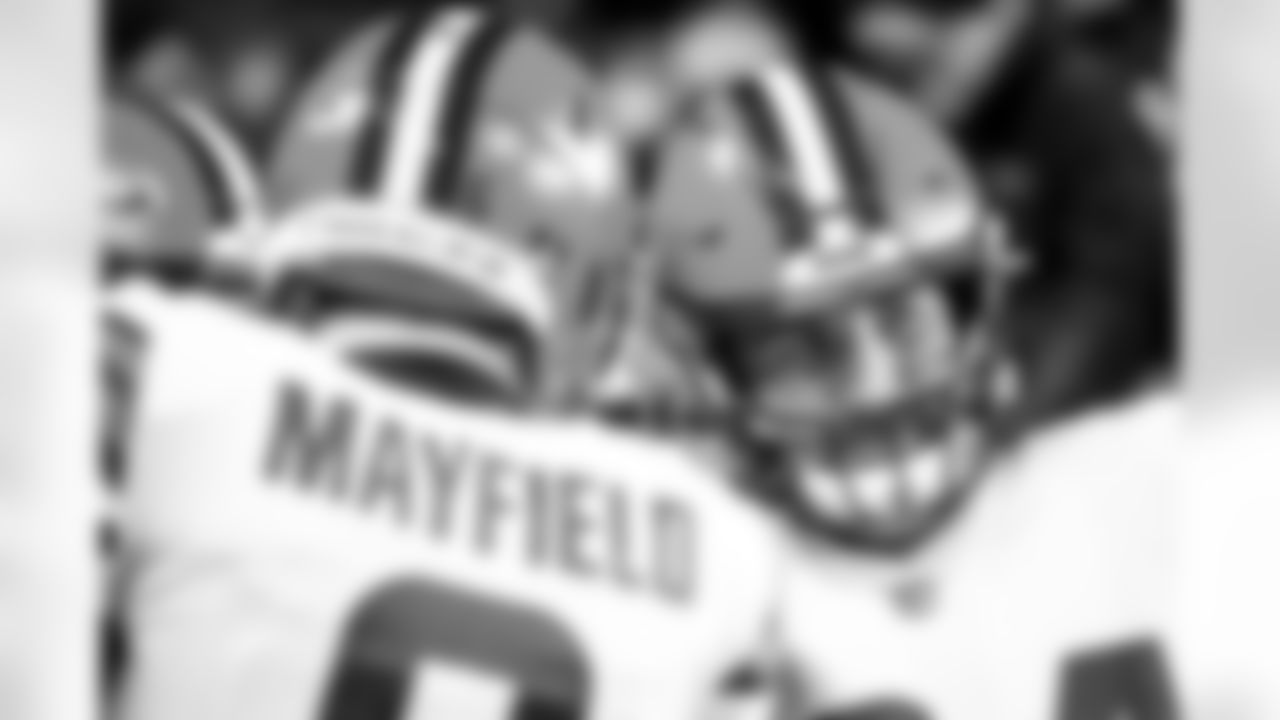The image is a low-quality, extremely blurry, black-and-white photograph that focuses on two football players. The player on the left, whose back is towards the camera, has "Mayfield" on his white jersey. The helmet of this player, difficult to discern in color due to the grayscale, features a distinct stripe pattern: a white stripe flanked by two thinner black stripes. The player on the right, facing the camera, has an indistinguishable face due to the blur. However, his helmet shares the same stripe pattern, and his jersey number is partially visible; one digit has a rounded top, and another seems to be a four but is also cut off. The image is zoomed in on these two players, who appear to be very close to each other, possibly touching or preparing for a collision. The background reveals a few additional football players, though they are merely indiscernible shapes. Overall, the photograph gives a sense of intense focus on the two main subjects amidst a hazy and unclear backdrop.